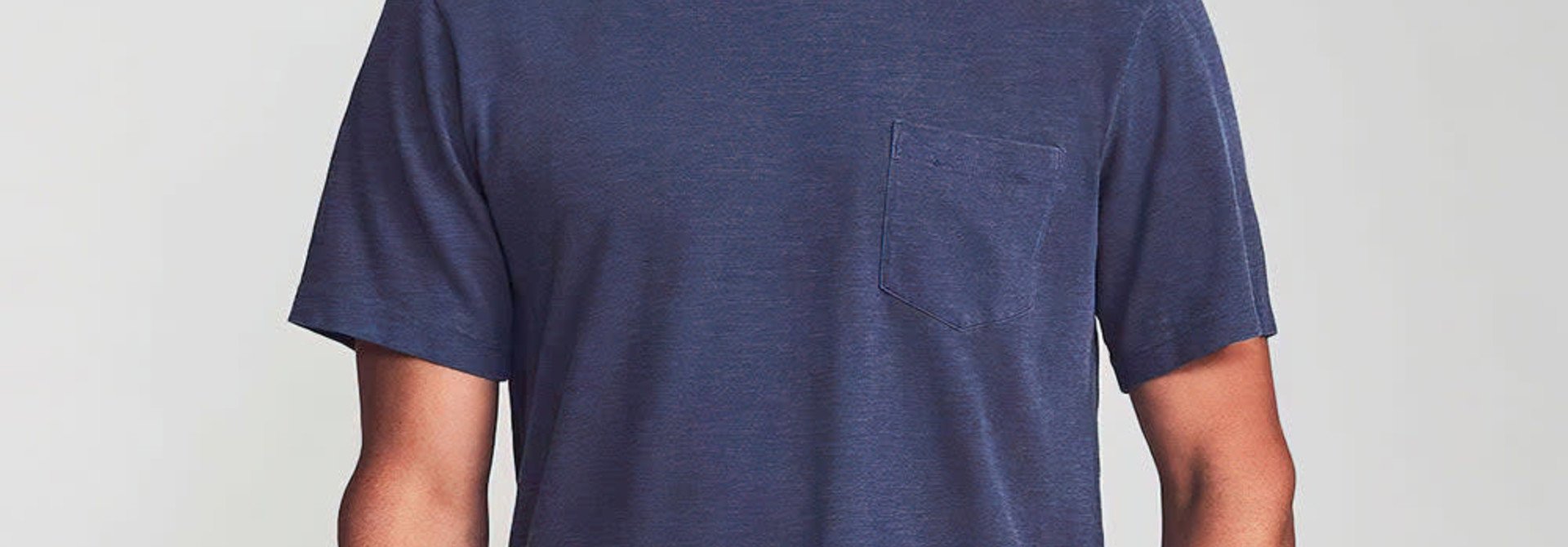This small, horizontal, rectangular image captures the chest area of a slender man, highlighting his dark blue, short-sleeve cotton t-shirt. The background is a light gray, creating a neutral setting that suggests a studio environment. The t-shirt features a pocket on the left side, above the chest. The shirt, while largely wrinkle-free and appearing freshly laundered, has some natural folds due to the man's slender build, causing it to hang loosely. The fabric exhibits a subtle distressed pattern, revealing hints of white within the dark blue fibers. The man's arms extend downward, showing the inside of his elbows, though the image cuts off before showing his hands and head. The model seems to have medium-toned skin, enhancing the visibility of the t-shirt against the plain gray backdrop, making the image suitable for a flyer or website advertisement.